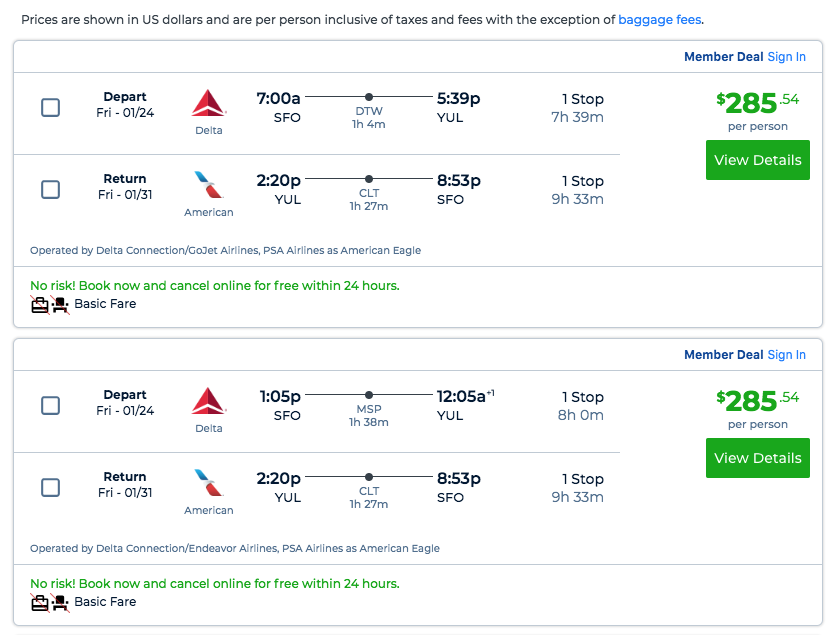This image, taken from a flight booking website, features a clean, all-white background with a structured layout. 

At the very top, there's a disclaimer in black text that reads, "Prices are shown in US dollars and are per person, inclusive of taxes and fees with the exception of" followed by "baggage fees" in blue text.

Below this disclaimer is the first rectangle, bordered in black. Inside this rectangle, there's a small white rectangle on the right side, outlined and featuring "Member Deal" in dark blue, followed by "Sign In" in light blue. A black line separates this section from the main content.

Within the main section of this rectangle, two different flights are listed. Each flight listing follows a consistent format. On the left side, each flight has a black-outlined square with white interior, stacked one above the other. 

Details for each flight start with the departure date at the top and the return date at the bottom. The airline for the outbound and return flights is listed next to the departure and arrival times, along with the total travel duration and information on any stops.

On the right side, under the "Member Deal Sign In" section, the price is prominently displayed as $285.54 per person. A large green button labeled "View Details" is positioned nearby.

Additional information under the return date indicates the operating airlines, such as "Delta Connection/Go Jet Airlines" and "PSA Airlines as American Eagle." 

At the bottom of each flight listing, there are notes in green stating, "No risk - Book now and cancel online for free within 24 hours." Details about the fare type are also included, specifying that it is a "Basic fare with no luggage, no seat attached."

Another flight is listed beneath the first with the same structured format and information.